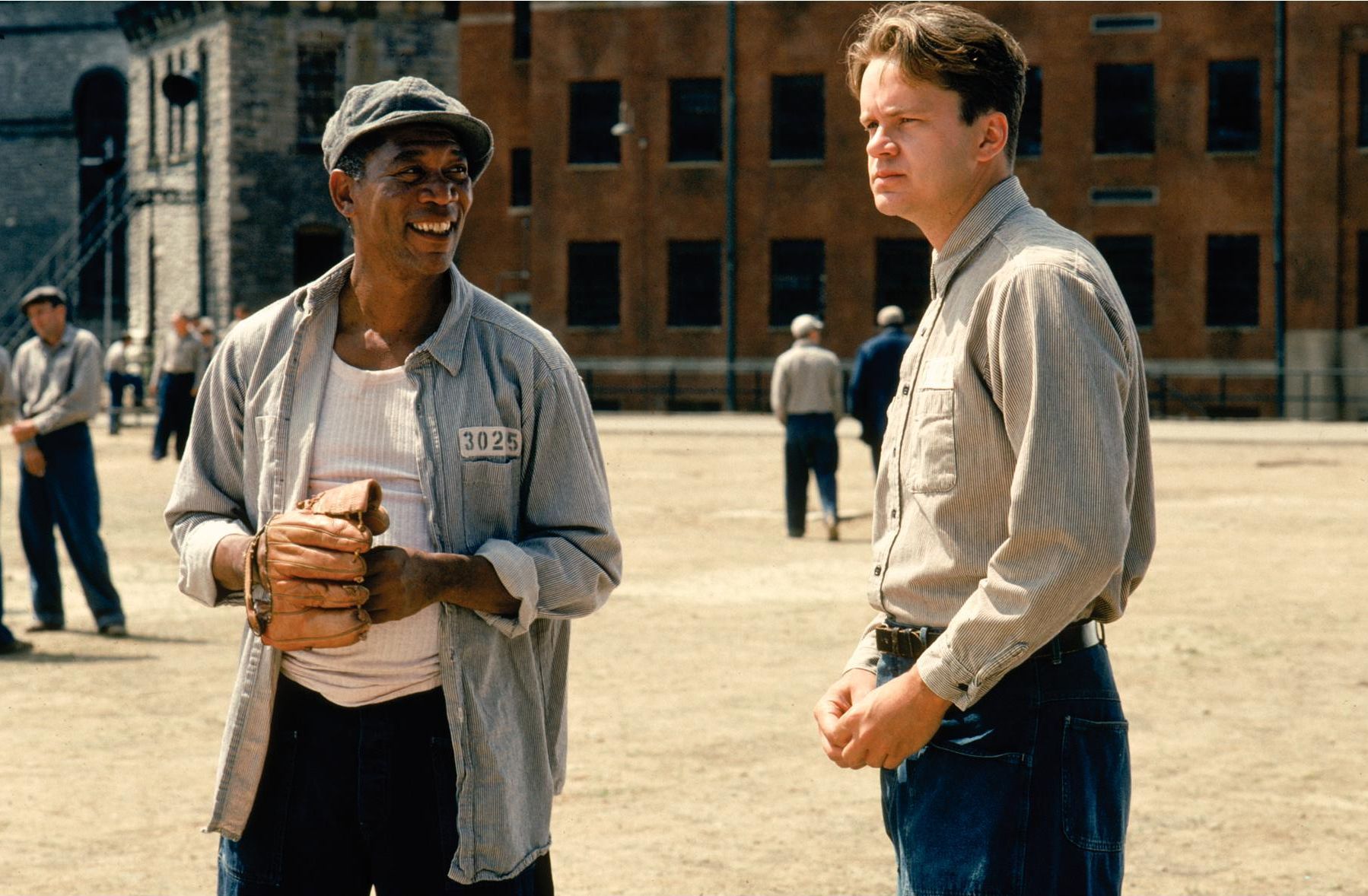In this still frame from the movie "The Shawshank Redemption," Morgan Freeman, portraying the character Red, stands on the left wearing a loose, unbuttoned blue long-sleeve shirt over a white t-shirt, blue pants, a short-brimmed blue cap, and a baseball glove on his right hand. His inmate number 3025 is visible on his shirt. Facing slightly to the right, Red is flanked by Tim Robbins as Andy Dufresne on the right, who is wearing a tucked-in gray shirt, blue jeans, and a belt. Andy faces to the left with his hands down in front of him. They are in a sandy dirt-covered prison yard, surrounded by other inmates in similar attire. Visible in the background are a red brick building with numerous windows and a stone building, indicating the prison complex.